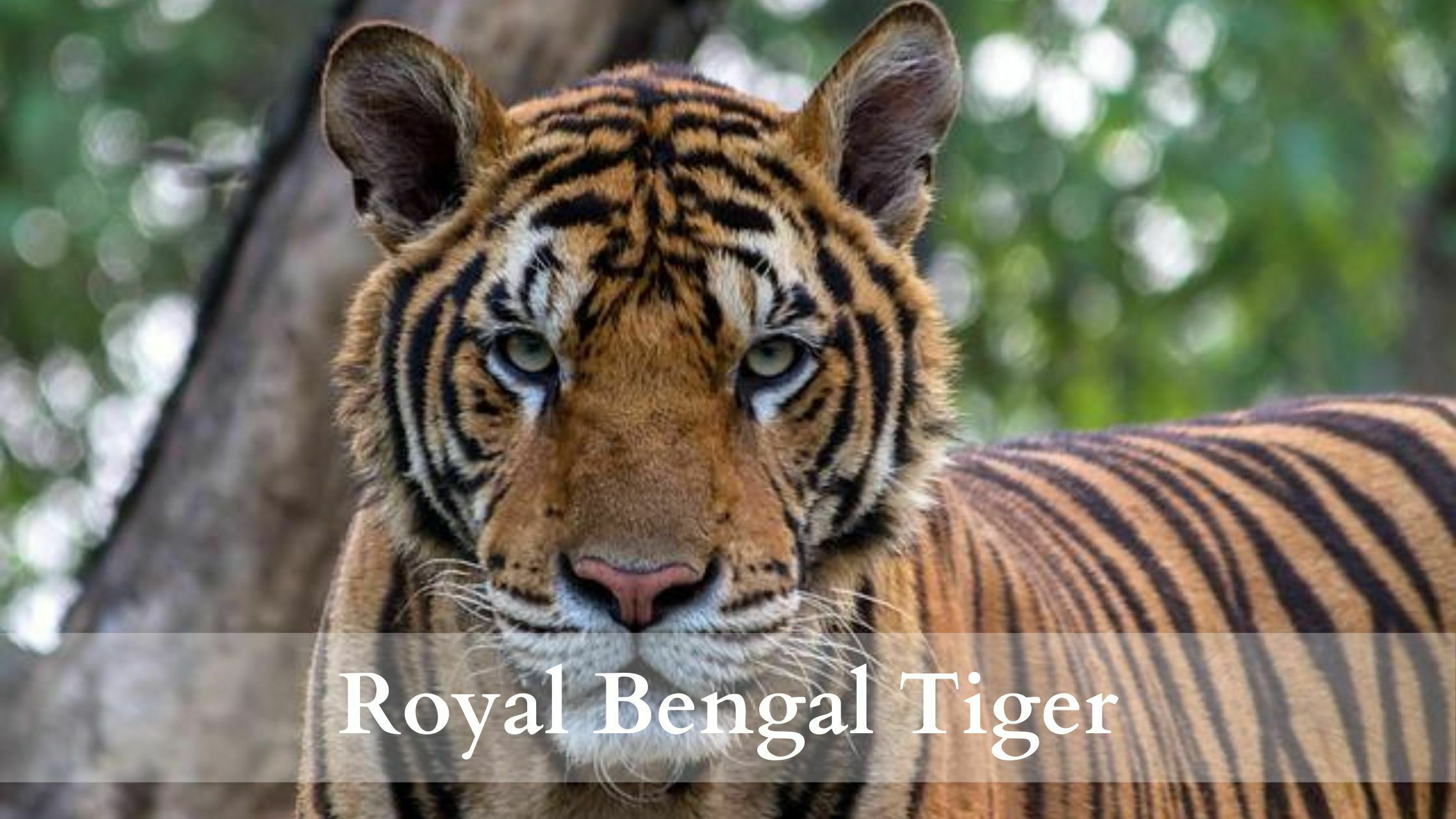The photograph captures the striking image of a Royal Bengal Tiger in the foreground, its powerful presence dominating the frame. This magnificent tiger, showcasing a typical orange coat with bold black stripes, stares directly at the camera with mesmerizing hazel-green eyes. White fur accents its face, encircling its eyes and mouth, while delicate whiskers sprout from its snout. Its nose is a soft, pale pink, adding an extra touch of detail to its regal visage.

In the background, soft-focus foliage and trees create a lush, blurred backdrop, emphasizing the tiger's prominence in the image. A translucent banner across the bottom of the photograph discreetly holds the white serif text, "Royal Bengal Tiger," identifying the species. This composition seems designed for digital use, perhaps on a website, where the text subtly informs without detracting from the tiger's visual impact. Despite the tiger's somewhat youthful appearance, its size and gaze convey a powerful, commanding presence.